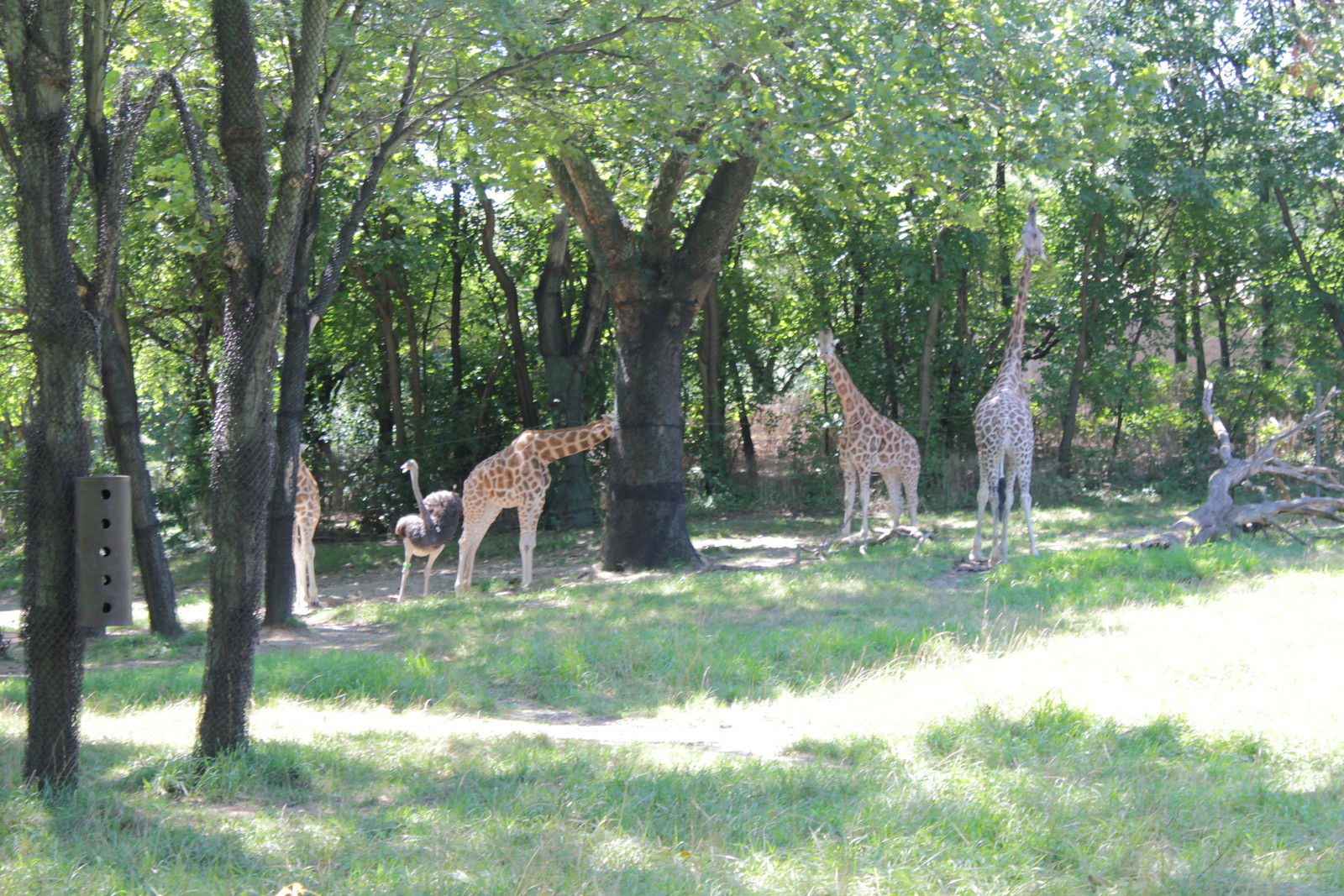This detailed color photograph captures a tranquil, shady grove within a zoo enclosure, likely in the northeastern United States. The scene is dominated by thick deciduous trees, their canopies creating a dappled sunlight effect on the grassy ground below. Amid the greenery, four giraffes are visible, each positioned differently. One giraffe stands with its head stretched high, possibly nibbling on leaves, while another appears to be chewing on tree bark. To the left, a giraffe's head peeks around a tree, making it difficult to discern whether it's facing forward or backward. Yet another giraffe looks toward the camera, distinguishable by its long neck and distinctive dark brown and light brown spots. 

Additionally, a large ostrich is present, with its black and white feathers slightly ruffled as if preparing to stretch its wings. The background showcases a fallen tree trunk, its branches sticking out amid the dense foliage, further enhancing the naturalistic setting. Not far from this fallen tree, a peculiar wooden object with five round holes is attached to a tree, possibly serving as a birdhouse or bat house. The lush greenery is interspersed with patches of bare earth, creating a rich tapestry of textures and colors in this serene zoo habitat.